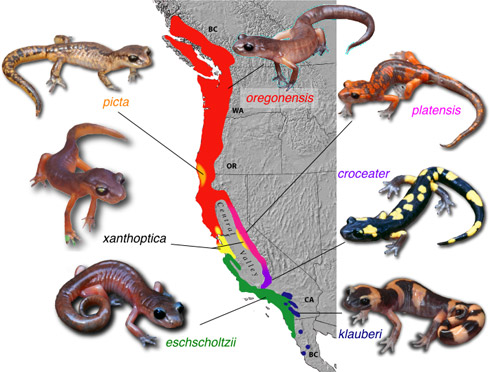The image features a detailed geographical and biological map of the western United States and southwestern Canada, spanning from British Columbia down to Southern California. The map is color-coded with regions in red, blue, green, purple, and yellow, highlighting various habitats. Superimposed on the map are seven different lizard species, each illustrated with vibrant colors: some are orange, some tan, one is dark blue with yellow spots, and another has orange and black stripes. These species include names like Oregonensis, Picta, Plutensis, Xanthoptica, Astrocia (Escholtzii), Clawberry (Klaubery), and the croc-eater. Lines connect each lizard to specific regions where they are found, providing a vivid depiction of their primary habitats across the mapped areas. The image also includes faint state borders and abbreviations such as B.C., W.A., O.R., and C.A., helping to identify the locations within the map.